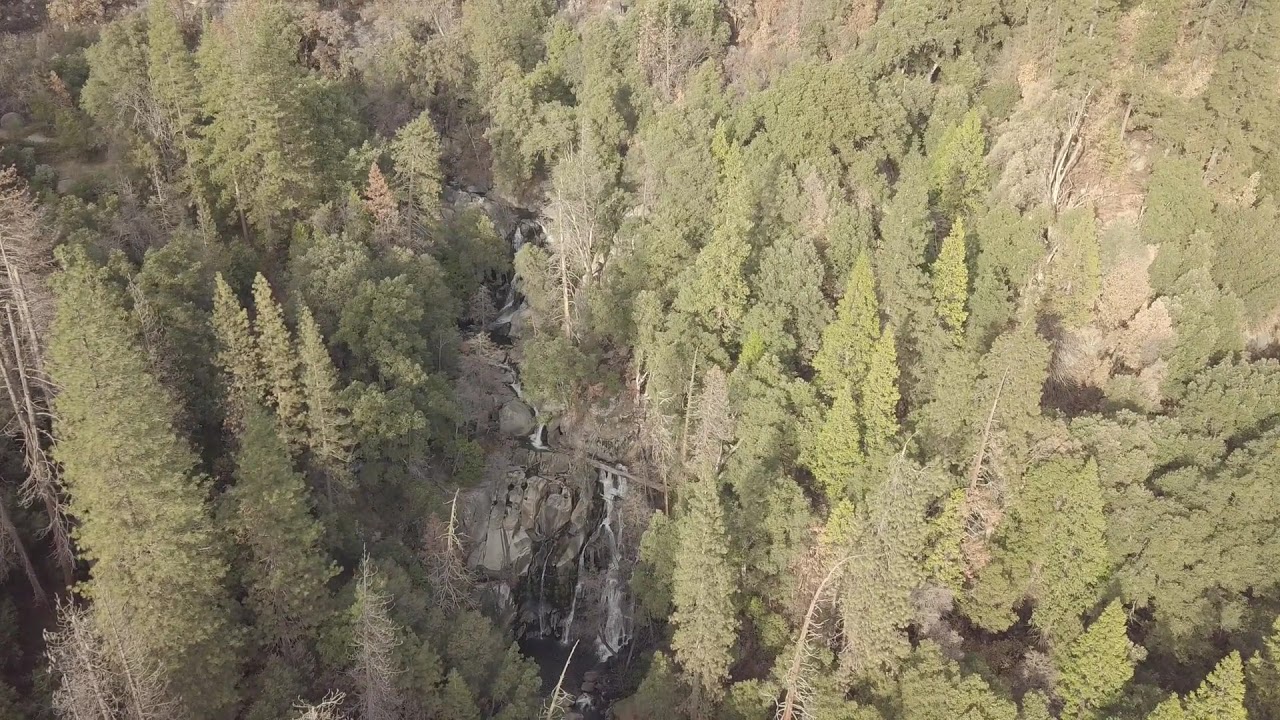An aerial photograph captures a sprawling forest, predominantly composed of various species of green, evergreen trees, mixed with other types of trees displaying vibrant shades of green, yellow, and some brown tones. The image, taken from a high vantage point, possibly from a helicopter, provides a clear view of the full structure of these trees, emphasizing their lush foliage. The scene is set on a bright, sunny day, with sunlight casting playful shadows throughout the landscape. In the center of this rectangular image, there is a prominent rocky cliffside, from which a series of small waterfalls cascade down, eventually cascading into a pool below. The rough, mountainous terrain interspersed with rocks adds to the natural beauty and suggests an inviting location for exploration or hiking. Despite the photograph's slightly off-color balance and limited quality, the dynamic interplay of flowing water and dense greenery creates a picturesque and serene setting.